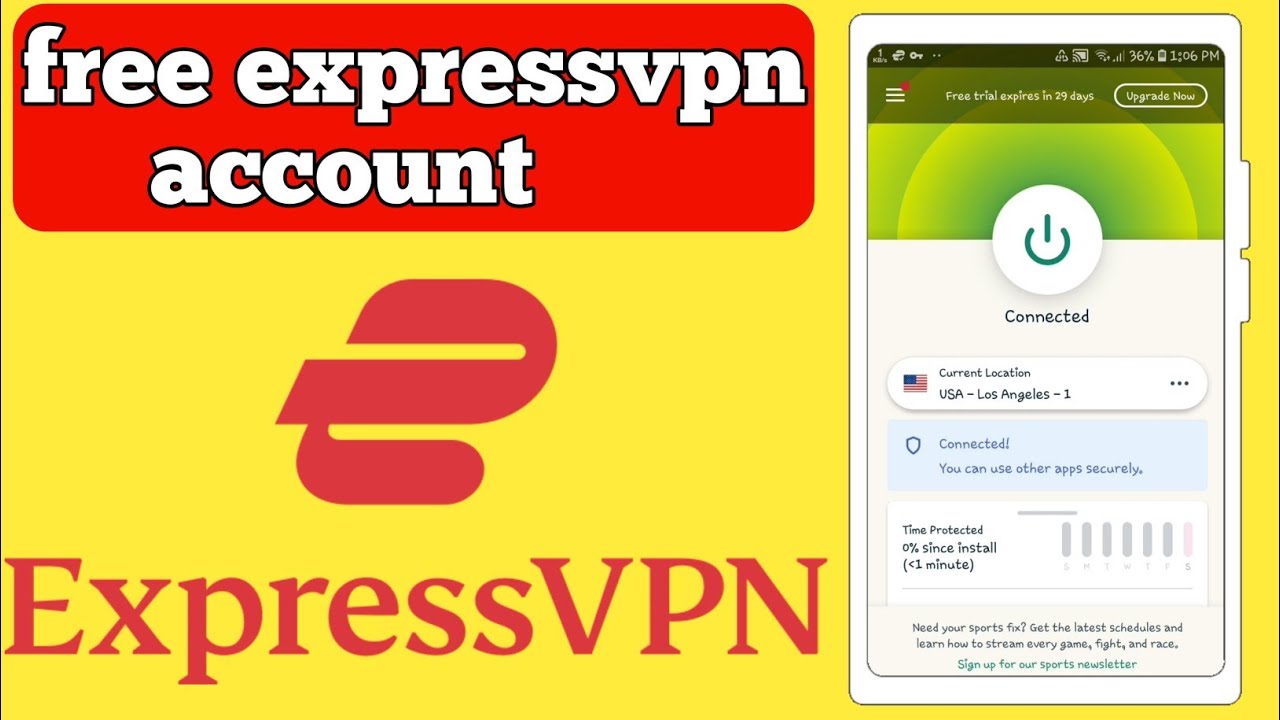The advertisement for the VPN service, ExpressVPN, showcases a sleek and simple design with a prominent yellow background. At the top, the white text reads "free expressvpn account" in all lowercase letters, drawing attention to the offer's exclusivity. Beneath it, in bold red text, the brand name "ExpressVPN" stands out.

To the right of the text, there is a detailed mock-up of the ExpressVPN application displayed on a mobile device. The device screen indicates it is 1:06 PM with a 36% battery charge, and it is connected to both cellular service and Wi-Fi. The interface of the ExpressVPN app shows a bright green "Connected" icon, confirming the current connection to a server located in Los Angeles, USA 1.

The app interface mentions that the free trial expires in 29 days with an option to "upgrade now." It highlights that the user can securely use other apps and indicates "time protected: under a minute," suggesting the app was just installed. Interestingly, there is also an option to sign up for a sports newsletter, diverging slightly from the main product focus.

Surrounding these elements, the advertisement’s vibrant colors and clear typography successfully convey the essential details and benefits of using ExpressVPN, making it an eye-catching and informative piece.